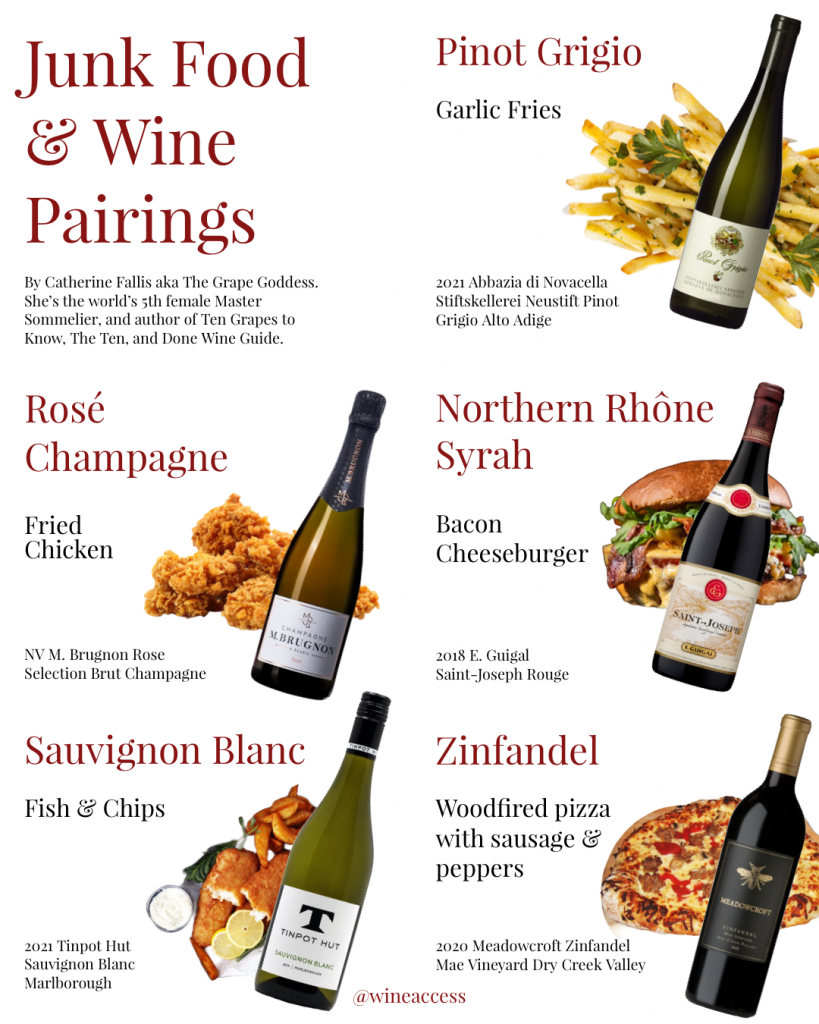This is a detailed guide on junk food and wine pairings presented on a clean, white background in burgundy lettering. Authored by Catherine Phallus, also known as the Grape Goddess, who is the world's fifth female master sommelier and author of "Ten Grapes to Know, the Ten and Done Wine Guide." The poster, titled "Junk Food and Wine Pairings," visually illustrates and notates six sections, each highlighting a specific wine paired with its ideal junk food companion.

At the top left, Rosé Champagne is paired with fried chicken, showcased with a bottle of Bergenon Rosé Selection Brut Champagne beside crispy chicken nuggets. Next, a bottle of 2021 Tin Pot Hut Sauvignon Blanc Marlboro is matched with a plate of classic fish and chips. On the top right, a 2021 Abbazia di Novacella Pinot Grigio Alto Adige complements a serving of garlic fries garnished with herbs. Below that, the 2018 E. Guigal St. Joseph Rouge Northern Rhone Syrah is the perfect match for a decadent bacon cheeseburger. Finally, at the bottom right, a 2020 Meadowcroft Zinfandel May Vineyard Dry Creek Valley is paired with a wood-fired pizza topped with sausage and peppers.

The poster includes detailed images of each food and wine pairing for easy visual reference, all curated by Catherine Phallus, emphasizing the harmony between popular junk foods and distinguished wines.